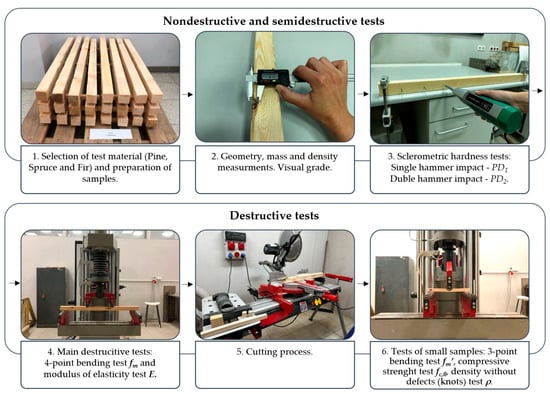The photograph displays a comprehensive instructional series of diagrams illustrating non-destructive, semi-destructive, and destructive testing procedures for wood samples. At the top, it is labeled "Non-Destructive and Semi-Destructive Tests," and comprises three images: 

1. The first image shows a selection of test materials, including stacks of pine, spruce, and fir wood, under the header "Selection of test material, preparation of samples."
2. The second image depicts an individual measuring a wooden plank using a device, with the label "Geometry, mass, and density measurements, visual grade."
3. The third image features a hand using a tool to perform a hardness test on the wood, captioned "Sclerometric hardness test, single hammer impact PD, dual hammer impact PD."

The lower section labeled "Destructive Tests" consists of three additional images:

4. The first image highlights the "Main destructive test, four-point bending test, and modules of elasticity test," showing a piece of wood subjected to pressure in a machine.
5. The second image shows a large cutting saw labeled "Cutting process."
6. The third image presents a piece of wood being tested in a machine, with the label "Test of small samples, three-point bending test, compressive strength test, density without defects test."

Each image and accompanying label meticulously details various testing methodologies for assessing the physical properties and performance of wood samples.